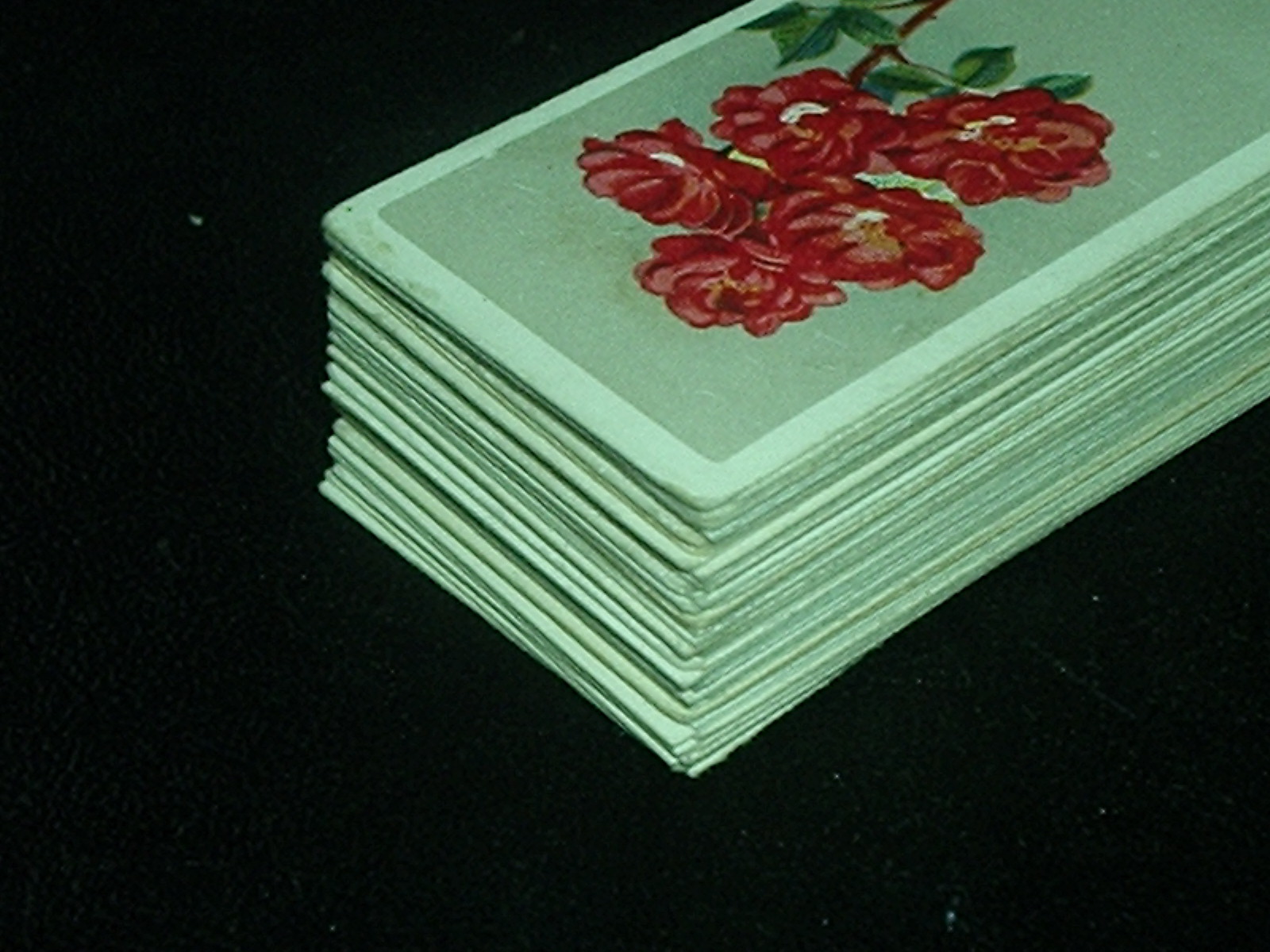The photograph captures a stack of mint green papers or cards set against a stark black background. Each item in the stack appears to be identical. The top card features an intricate design: it has a thin, light green border approximately a quarter to half an inch wide, framing a darker green interior. Within this darker section, there is a detailed painting of fully bloomed red roses with white centers. The flowers are depicted with wild, naturalistic charm, showcasing brown stems adorned with thorns and lush green leaves. The edges of the stack are slightly uneven, giving a jagged appearance as the cards do not perfectly align.